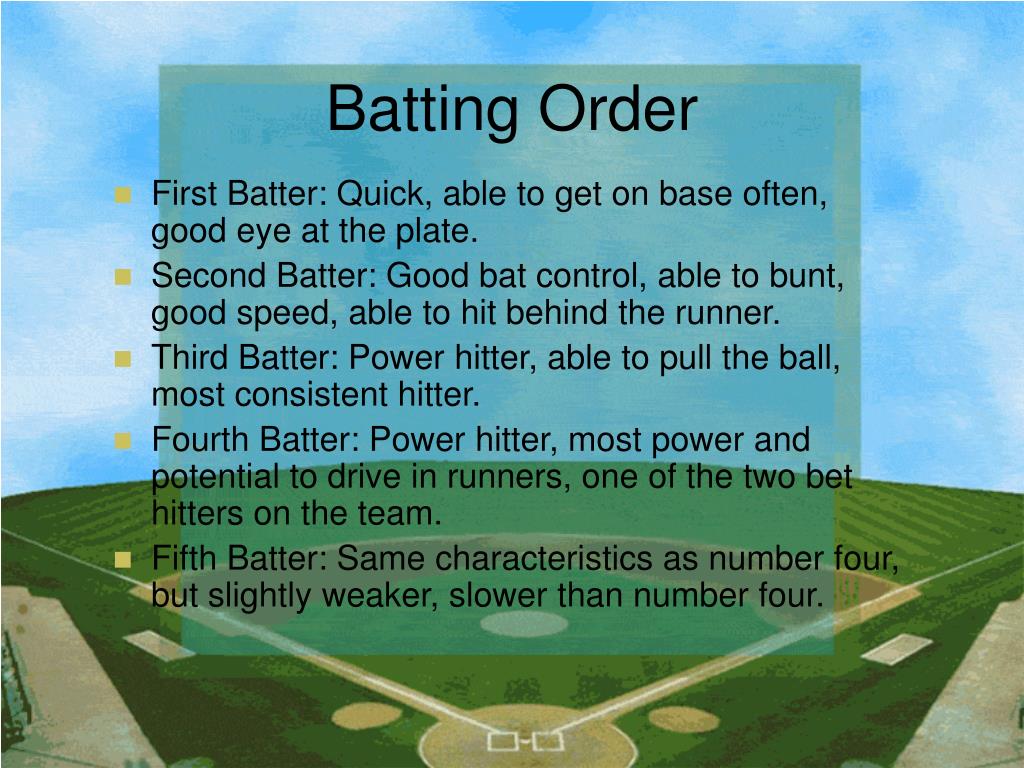The image features a well-manicured baseball field as its background, complete with bases clearly visible, extending from the bottom to the middle section of the frame. Above this, the sky forms the upper part of the scene, lending depth and context to the setting. Dominating the foreground is a large block of text, detailing a batting order. The text, written in shades of white, blue, turquoise, black, green, and tan, is meticulously organized, making it easy to read. It serves an educational purpose for sports enthusiasts, providing detailed characteristics of each batting position: 

1. First batter - quick, able to get on base often, with a good eye at the plate.
2. Second batter - exhibits good bat control, adept at bunting, has good speed, and can hit behind the runner.
3. Third batter - a power hitter, able to pull the ball, and is the team's most consistent hitter.
4. Fourth batter - the one with the most power and potential to drive in runners, considered one of the two best hitters on the team.
5. Fifth batter - shares similar characteristics with the fourth but is slightly weaker and slower.

The overall composition places emphasis on the textual information, suggesting the image's use as an educational tool for those interested in the sport of baseball.